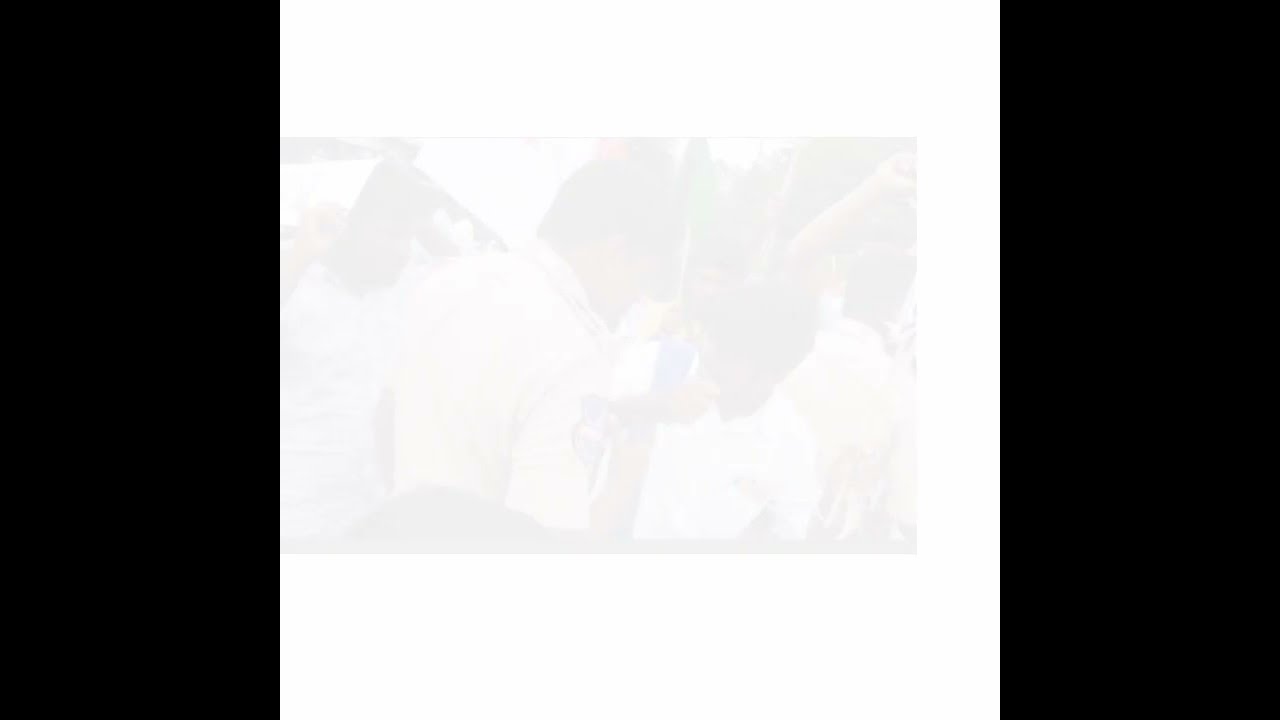The image features a central, almost indistinguishably faded photograph, set against a stark, white background. The photograph, in a portrait orientation, appears to depict an adult leaning toward a child, possibly engaging in conversation, with other figures faintly visible in the backdrop. They all seem to be outdoors, perhaps dressed in white shirts, but the details are incredibly blurry and difficult to discern. Framing this central white area are two solid black rectangles on the left and right sides, creating a landscape orientation for the overall image. The black bars serve as borders, emphasizing the white background and the nearly ethereal quality of the faint photograph within. The extreme fading of the photo gives it a mysterious and indistinct quality, making it challenging to interpret the exact nature of the scene.